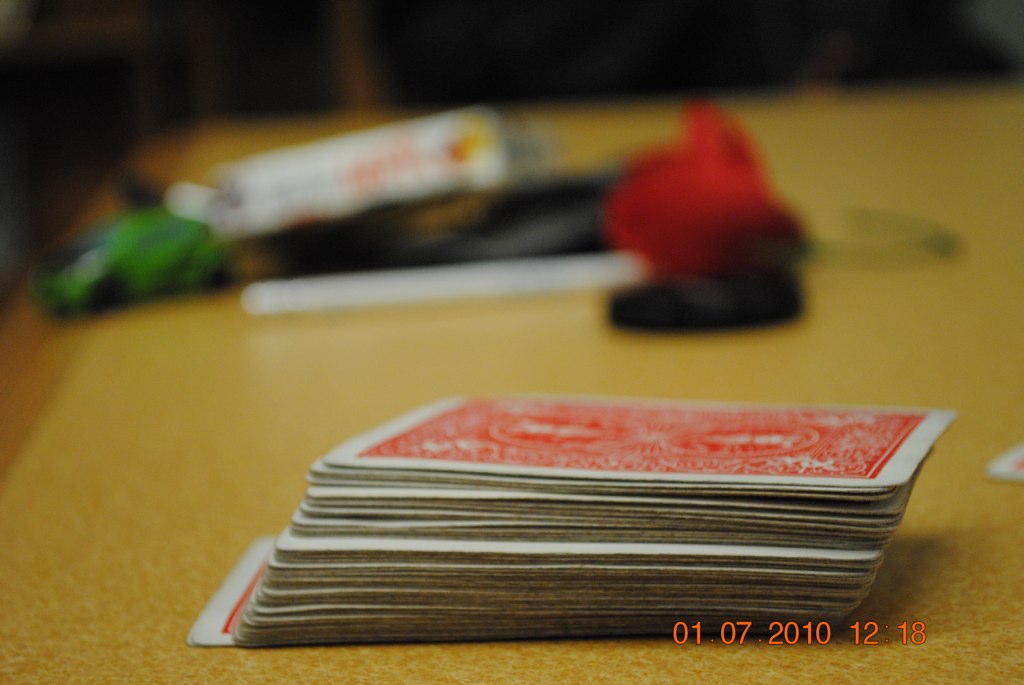A highly detailed image depicts a deck of cards placed centrally on a brown dining table. The deck, featuring a red background with intricate white floral and wavy patterns, is the main focus of the picture. 

In the background, several items can be seen. To the left, there is a plastic rose with red petals and a green, wire-like stem bent into a U-shape, resting on what appears to be a black remote control. Just beyond the rose, a book with a black cover is visible, topped by a box adorned with red and yellow writing. In the top-left corner of the image, a green toy car with blue windows is positioned. 

The timestamp at the bottom of the image reads "01.07.2010 at 12.08.2010."